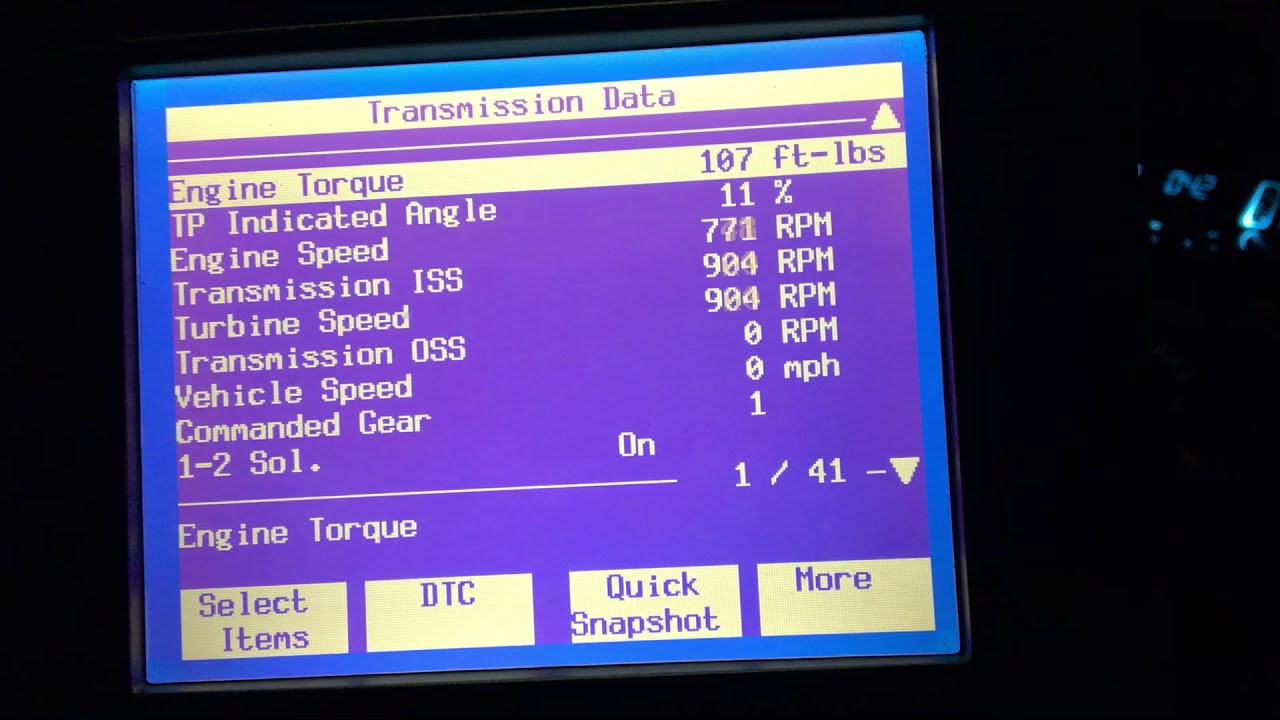This image features a detailed screenshot of vehicle diagnostic data on an LED screen. The screen has a predominantly dark or bright blue border and a purple center, with a white bar at the top displaying "Transmission Data" in purple letters. Below this header, various measurements and parameters related to engine and transmission performance are listed, including:

- Engine Torque: 107 ft-lbs
- TP Indicated Angle: 11%
- Engine Speed: 771 RPM
- Transmission ISS: 904 RPM
- Turbine Speed: 904 RPM
- Transmission OSS: 0 RPM
- Vehicle Speed: 0 MPH
- Command Gear: 1 (with 1-2 SOL marked as "On")

Additional on-screen options such as "Select Items," "DTC," "Quick Snapshot," and more are available. There are arrows pointing to various metrics, and four white squares are visible at the bottom. The numeral "042" is discernible behind the information, possibly indicating a specific data point or setting on the device. The dark background and blue lighting add to the high-tech appearance, suggesting this could be a specialized diagnostic tool used in vehicle maintenance or testing environments.